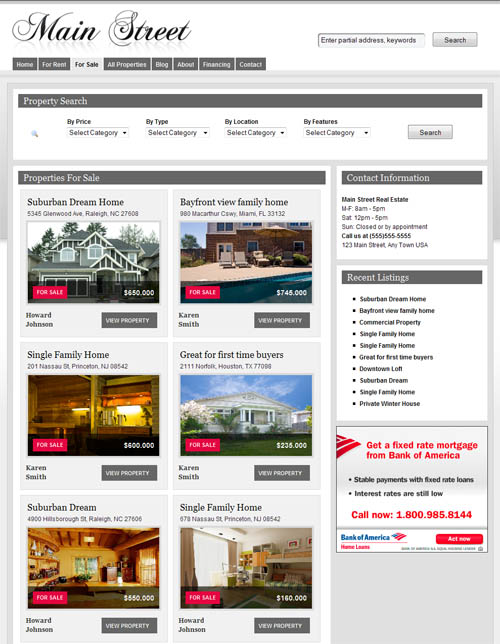A detailed caption for the given screenshot of a real estate listing site:

---

The screenshot displays a real estate listing website named "Main Street," prominently shown at the top in a cursive font. Below it is a search bar that invites users to "enter partial address, keywords" with a gray search button on the right. The site features a dark gray navigation menu at the top with several tabs including Home, For Rent, All Properties, Blog, About, Financing, and Contact. The "For Sale" tab is currently active and is highlighted in light gray.

A broader search panel below the navigation bar, labelled "Property Search," allows users to filter listings by price, type, location, and features. Six property listings are displayed in a grid format, with two properties per row over three rows:

1. **Suburban Dreamhouse**: This listing features a photo of a modern, gray, two-story house.
2. **Bayfront View Family Home**: The image displays a poolside setting with three beach chairs, suggesting the house is near the ocean.
3. **Single Family Home**: An interior shot bathed in yellow lighting, possibly showcasing a kitchen, though the specific room type is unclear.
4. **Great for First-Time Buyers**: Features a single-story house with a protruding porch and a clear blue sky in the background.
5. **Suburban Dream**: Shows an indoor kitchen area marked by wooden rafters and paneling, accentuated with warm yellow tones.
6. **Single Family Home**: Likely depicting a bedroom, or possible living space, with white walls, shelving, and an open window.

On the side, the layout includes columns with sections for contact information, recent listings, and an advertisement for a fixed-rate mortgage from Bank of America.